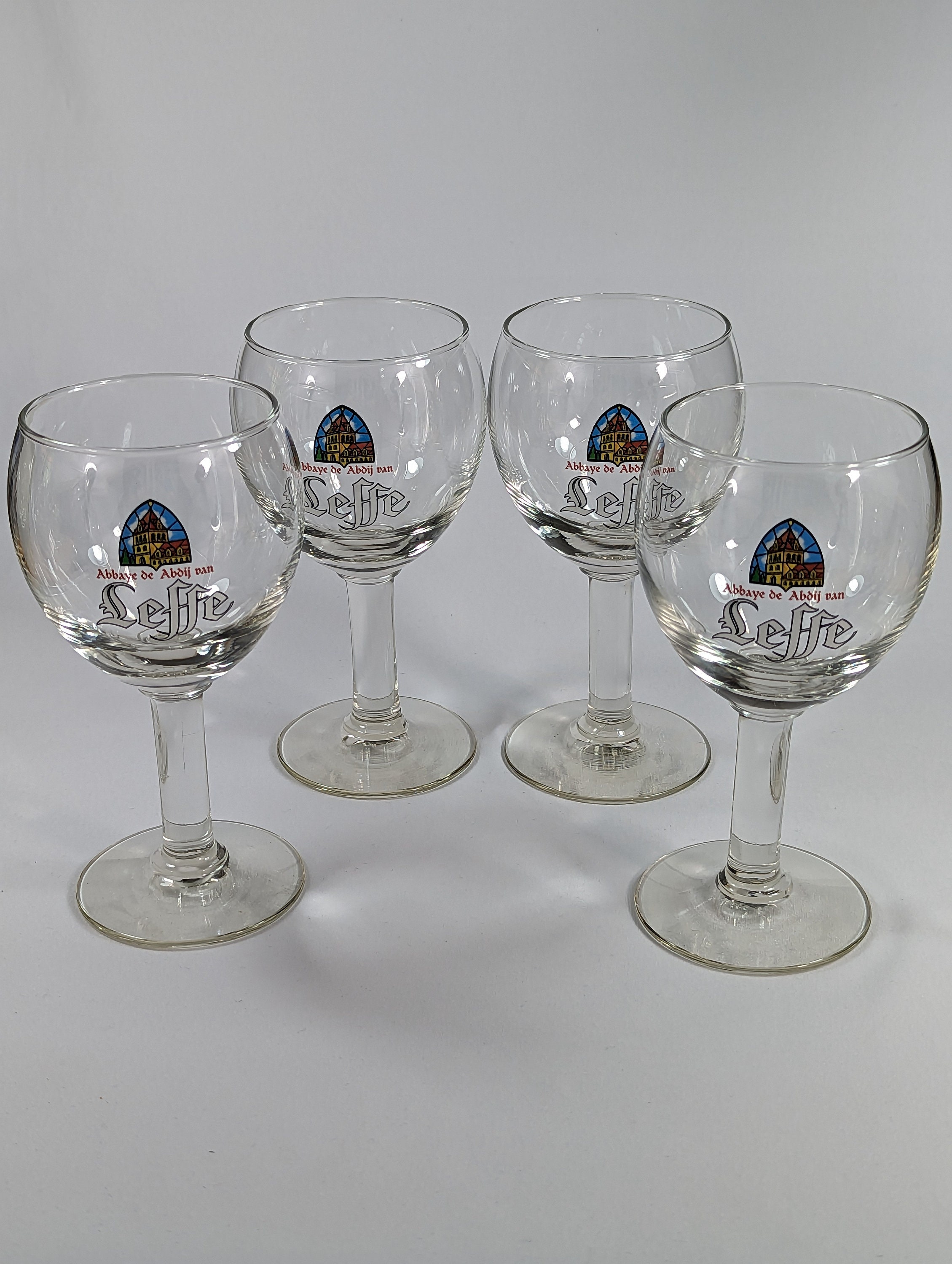The image depicts four identical wine glasses, constructed from glass, sitting on a gray countertop under artificial lighting in a vertically rectangular, full-color photograph. Each glass has a thick stem and a sturdy base, lending a fancier feel suitable for a nice drink, perhaps beer or wine. The glasses are adorned with a detailed design positioned above the word “LEFFE” in an old-style font. The design features a half-oval frame encompassing a blue sky and a brown building that resembles a church with stained-glass imagery, reinforcing a European aesthetic. The scene appears meticulously staged, devoid of borders, with a glowing light source highlighting the glasses against a subtle white and gray background.